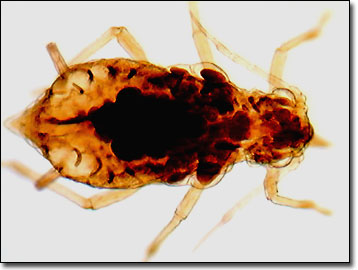The image features a detailed colored drawing of an insect, predominantly orange with black areas on its back and the center of its head. The insect has a distinctly round body with a smaller, circular head. Two long antennas extend from its head, positioned in front of its slightly translucent, bright eyes, accompanied by a single feeler. The insect also has two horn-like appendages on its back and six legs, which are yellowish and partially see-through. There are tiny wing-like structures near its neck, hinting it might be a bumblebee. The insect is depicted in an x-ray-like view, from an upper angle, making it appear as if viewed through a microscope. The background is white, enclosed by a thin black border, emphasizing the clarity and intricacies of the insect's form. The overall composition gives it a scientific, almost brain scan-like appearance.